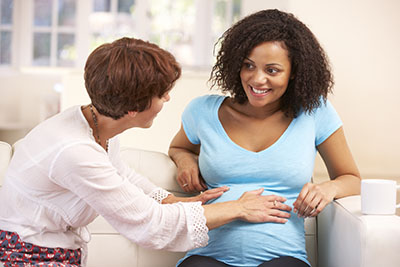The photograph captures a touching moment between two women in a cozy indoor setting, likely a living room. They are seated on a white sofa with a white mug placed beside them. The woman on the right has curly, frizzy hair that is somewhere between black and brown, and she is wearing a light blue t-shirt. Her rounded belly suggests that she is pregnant, and her chocolate-brown skin radiates a natural glow as she smiles warmly.

Beside her, the woman on the left sports short, reddish-brown hair and is dressed in a long-sleeved shirt that might be white or slightly pink, complemented by pants that feature a red and blue repetitive pattern. This woman is gently placing both her hands on the pregnant woman's belly, perhaps to feel the baby kicking. The affectionate gaze exchanged between them highlights their special bond. In the background, a cream-colored wall completes the scene, adding to the warmth and intimacy of the setting.